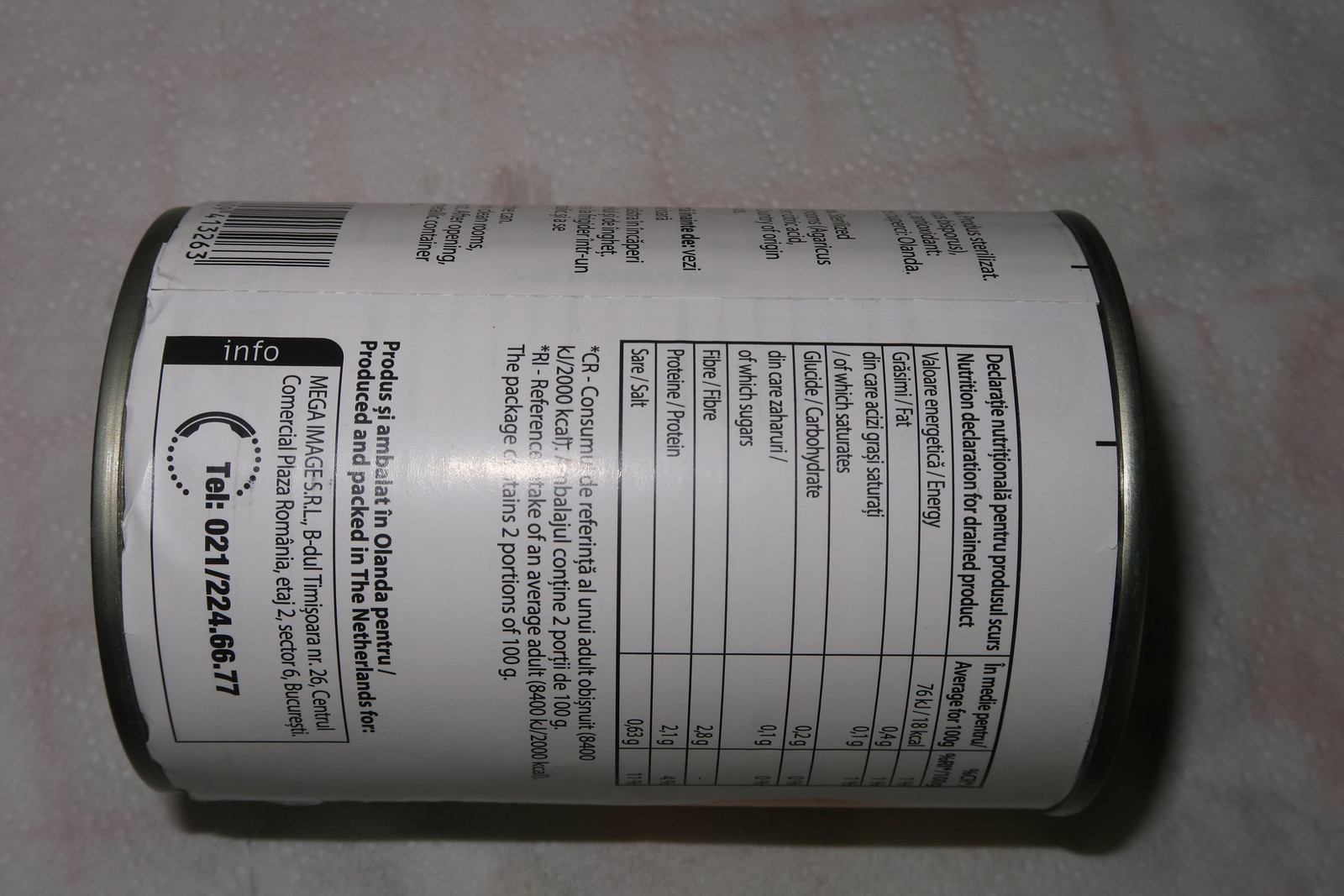This close-up photograph captures a canned food product, lying on its side on a checkered pink table or paper towel. The can features a prominent black and white label, detailing nutritional facts and other information. The label is primarily white with black printing, including a nutrition facts table and text beneath it. Below this section, there is a rectangular box displaying the manufacturer's address and a telephone number (Tel: 021/224.66.77), indicating the product was produced and packaged in the Netherlands for a company based in Bucharest. The label also contains an “info” sign and mentions "mega image" suggesting a brand or informational section. The nutrition information includes measurements in kilograms and details on fiber, protein, and energy content. The side view reveals details in Dutch, clarifying the product's origin.